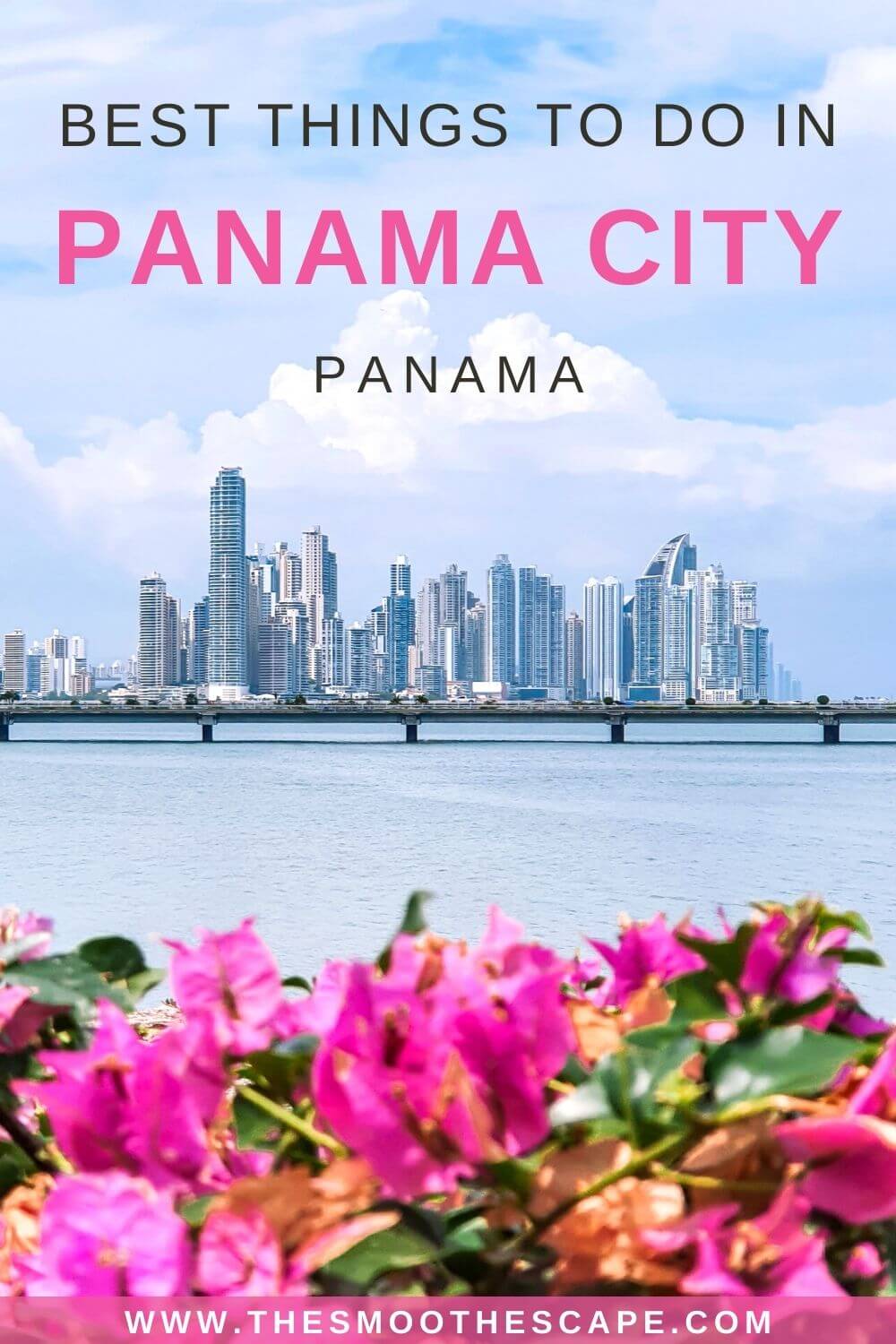This image captures a stunning view of Panama City, Panama, from across the bay. Spanning approximately three inches in width and six inches in height, the photograph features a brilliant blue sky adorned with fluffy white clouds. The foreground showcases vibrant pink tropical flowers with lush green leaves, framing the picturesque scene. A bridge, potentially for vehicular or pedestrian use, stretches partway across the water, adding an architectural element to the composition. The skyline of Panama City stands prominently in the background, highlighting its modern and inviting urban landscape. At the bottom of the image, the website www.thesmoothscape.com is displayed, suggesting that this photo serves as a promotional piece aimed at enticing travelers to visit Panama City, Panama.